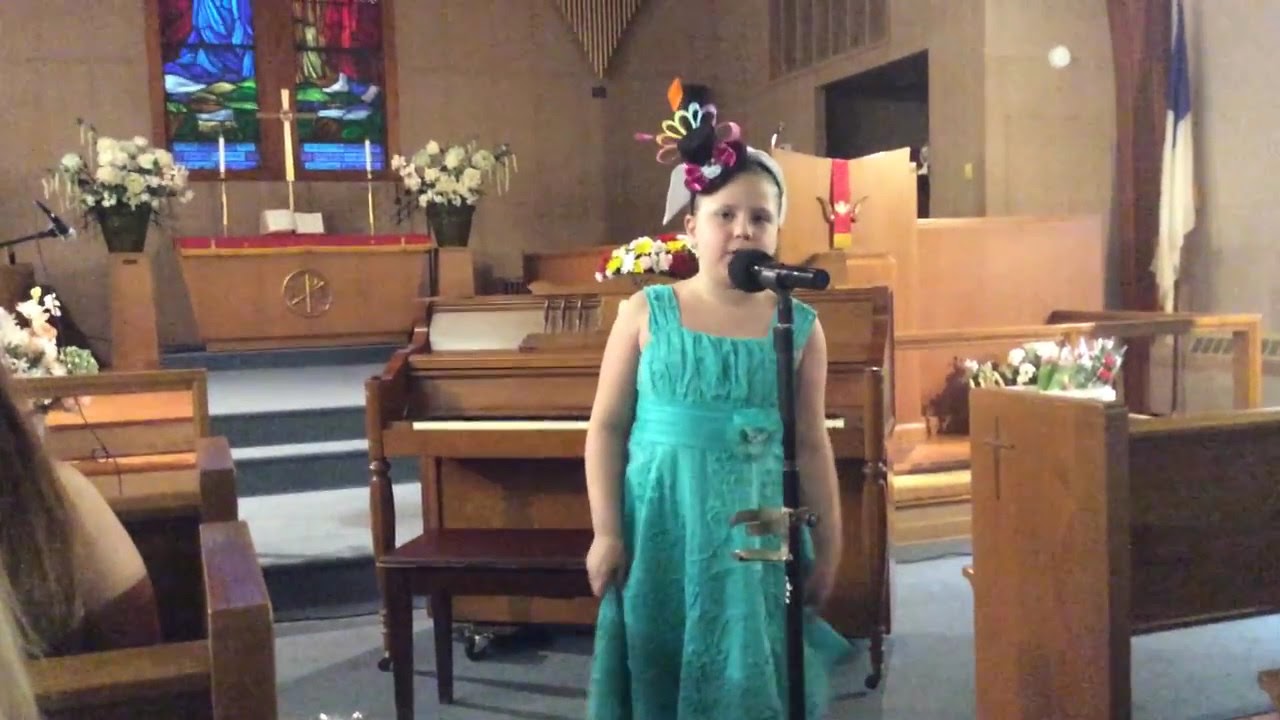In this horizontally aligned rectangular picture taken inside a church building, a young Caucasian girl is centered, standing at a black microphone, evidently singing or speaking. She appears to be around 10 years old and wears a sleeveless, aqua green dress with a lacy bottom and a flower detail around her waist. Her headpiece, a white headband adorned with a colorful flower with multicolored petals and a black center, adds a playful touch to her outfit.

The setting shows light brown wooden pews on either side of the girl. Notably, the pew on the right features a carved cross, while on the left, only the backside and right arm of a woman wearing a white top with long hair is visible. The altar area behind the girl features a wooden table with potted white flowers and candles arranged on either side. 

Further back, there's a piano or organ, and the brown walls are lined with stained glass windows in hues of red, blue, and green. The background is partially obscured as the picture cuts off, leaving the upper wall unseen. A white and blue flag is situated in the upper right corner, surrounded by more flowers positioned on the ground. The carpet in the image is a bluish-gray, contributing to the serene ambiance of the room.